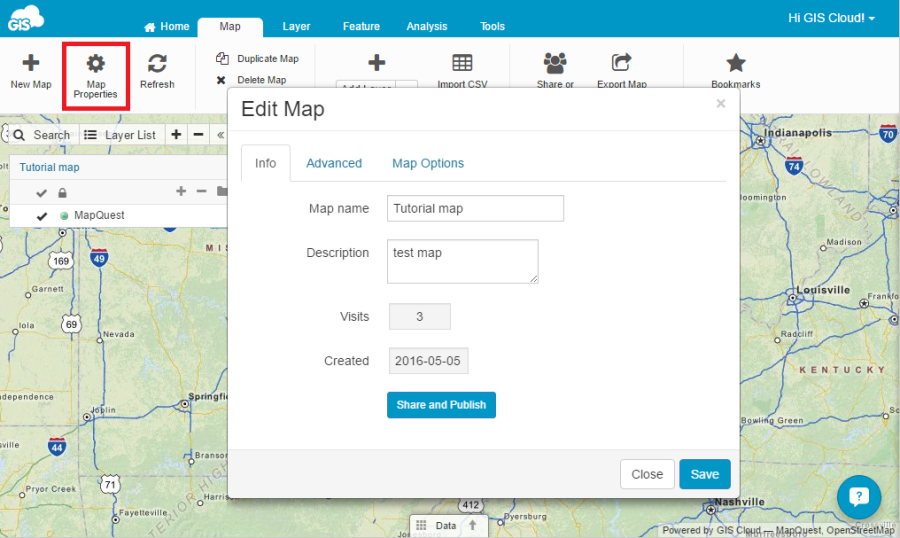**Image Description:** 

The image depicts a digital interface of a Geographic Information System (GIS) map, focused on the regions of Indiana, Kentucky, and parts of surrounding states. The upper left corner features the acronym "GIS" alongside an icon of a cloud. A blue navigation banner spreads across the top, containing menu options labeled "Home," "Map" (which is highlighted), "Layer Features," "Feature Analysis," and "Tools." Below this banner is another line displaying a button labeled "New Map," a gear icon, and the text "Map Properties" enclosed in a red border.

The central portion of the image showcases the map itself, although it is largely obscured by a large white square overlay. Visible portions of the map show parts of Indiana, Kentucky, Tennessee, and surrounding states. Notable cities marked on the map include Indianapolis, Madison, Louisville, Radcliffe, Bowling Green, Nashville, Garnet, Nevada (a city in Missouri), Fayetteville, and Pryor Creek.

Within the white overlay, the top left corner is labeled "Edit Map." Three tabs—"Info," "Advanced," and "Map Options"—are also visible. Beneath these tabs is a section titled "Map Name" with a text box populated with "Tutorial Map." Following this is the "Description" section containing the text "Test Map." Further down, it notes "Visits: 3" and "Created: 2016-05-05." At the bottom, two buttons are present: "Share" and "Publish."